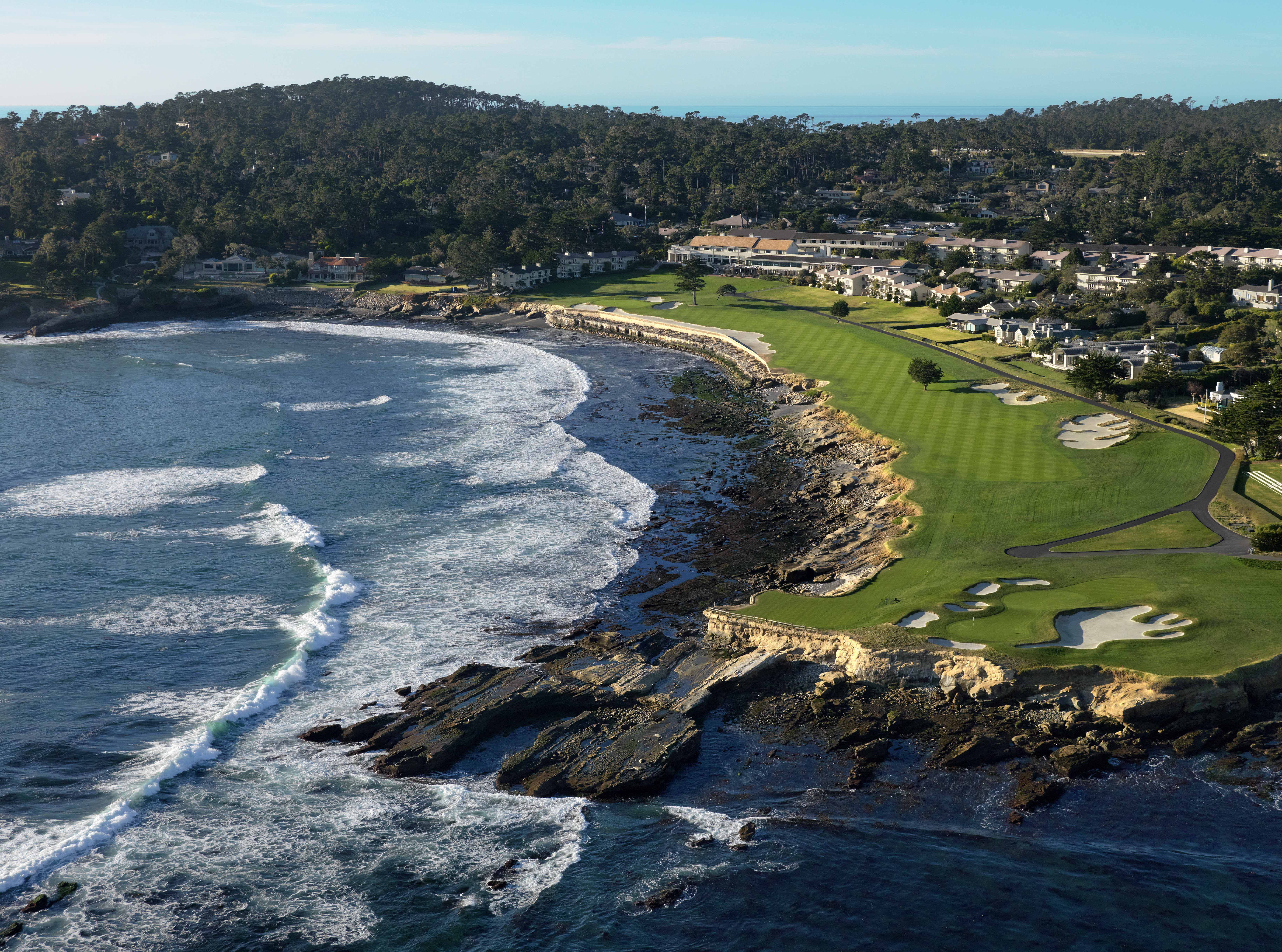This image beautifully captures an aerial view of a coastal golf course nestled where the rugged land meets the expansive sea. The lush green fairways and meticulously maintained putting greens of the golf course stand in striking contrast to the rugged rocky cliffs that line the edge of the shore. The deep blue ocean lies to the left of the frame, with waves that create a frothy white foam as they crash against the shoreline and rocks, adding to the scenic drama of the coastal landscape.

Several of the golf course's holes are positioned perilously close to the cliff's edge, offering dramatic views and challenging play. Sandy bunkers and neatly lined pathways crisscross the vibrant green expanse, while a scattering of trees adds a touch of natural beauty to the carefully curated landscape.

In the background, residential homes and structures blend harmoniously with the natural environment, their muted tones and surrounding trees creating a seamless transition from man-made to natural beauty. These houses are part of a larger development that extends across the horizon, framed by a slightly mountainous, forested region. At the very top of the image, the bright blue sky is dotted with a few light clouds, casting a bright sunlight over the scene and enhancing the overall picturesque quality of the view.